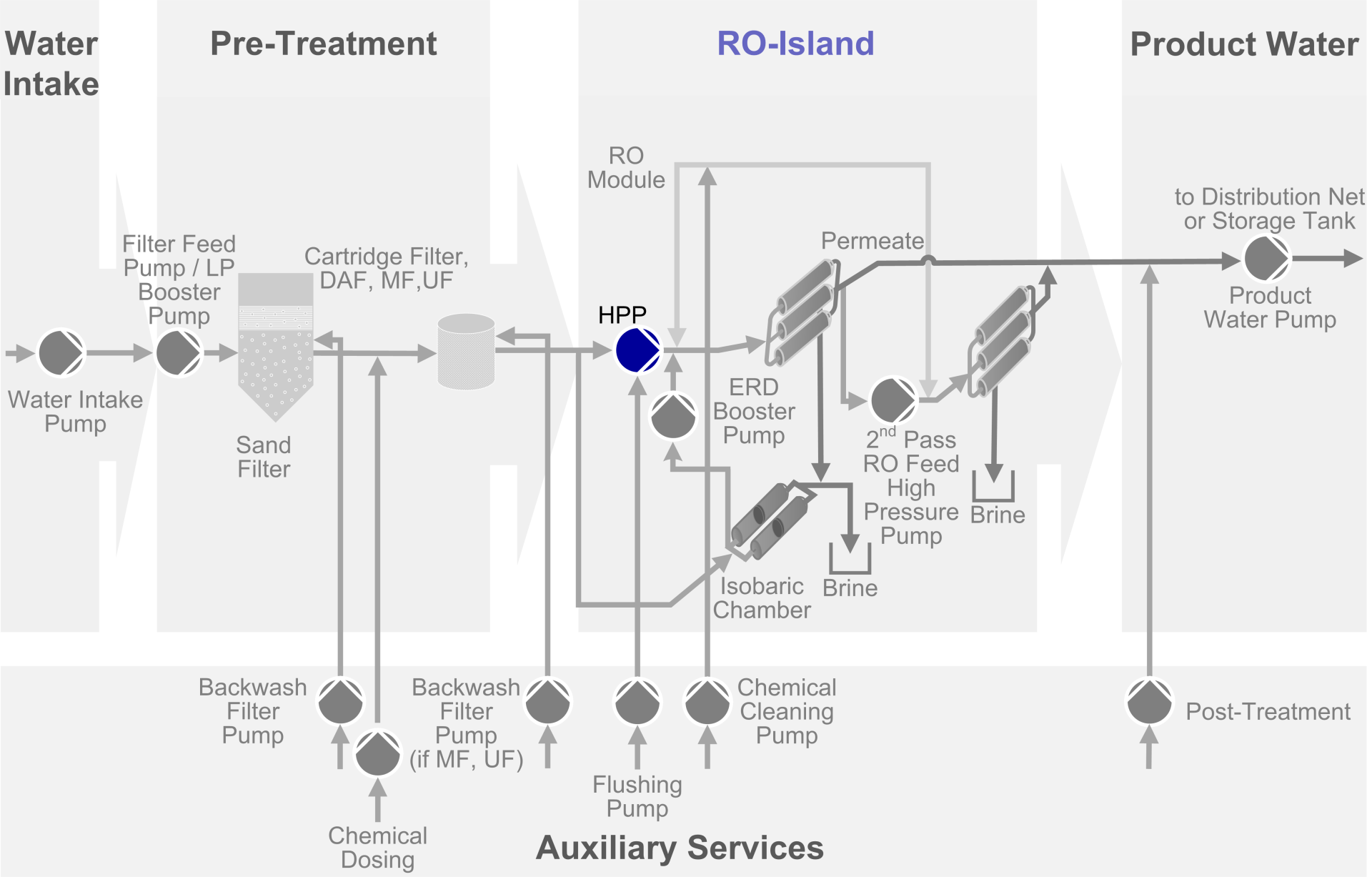This image is a detailed process diagram of a water treatment system, visually illustrating the journey of water from intake to product water. The diagram is laid out horizontally from left to right within translucent light gray boxes, each connected by arrows that guide the flow through various stages. The main stages are: Water Intake, Pre-Treatment, RO Island, and Product Water, with auxiliary services detailed below.

The diagram begins with the Water Intake section, showing a water intake pump directing water into the Pre-Treatment stage. This Pre-Treatment box includes components such as a cartridge filter, a sand filter, and a filter feed pump, each connected by arrows indicating the direction of water flow.

Next is the RO Island section which houses critical components including a high-pressure pump (HPP), an ERD booster pump, an RO (Reverse Osmosis) model, and an isobaric chamber. Blue labeling highlights the RO Island and the high-pressure pump, emphasizing their importance in the process.

Following the RO Island, the water moves into the Product Water section, where it can be directed either to a distribution net or to a storage tank with the help of product and water pumps.

Beneath the main process flow, Auxiliary Services are outlined in a long gray rectangle. This section includes elements like a backwash filter pump, chemical dosing systems, a flushing pump, chemical cleaning pump, and both NF (nanofiltration) and UF (ultrafiltration) units. These services support the main process by ensuring clean filters and proper chemical balances.

Overall, the diagram efficiently showcases the sequential steps and equipment involved in the water treatment process using arrows, gray circles, and labeled components within a light gray color scheme.